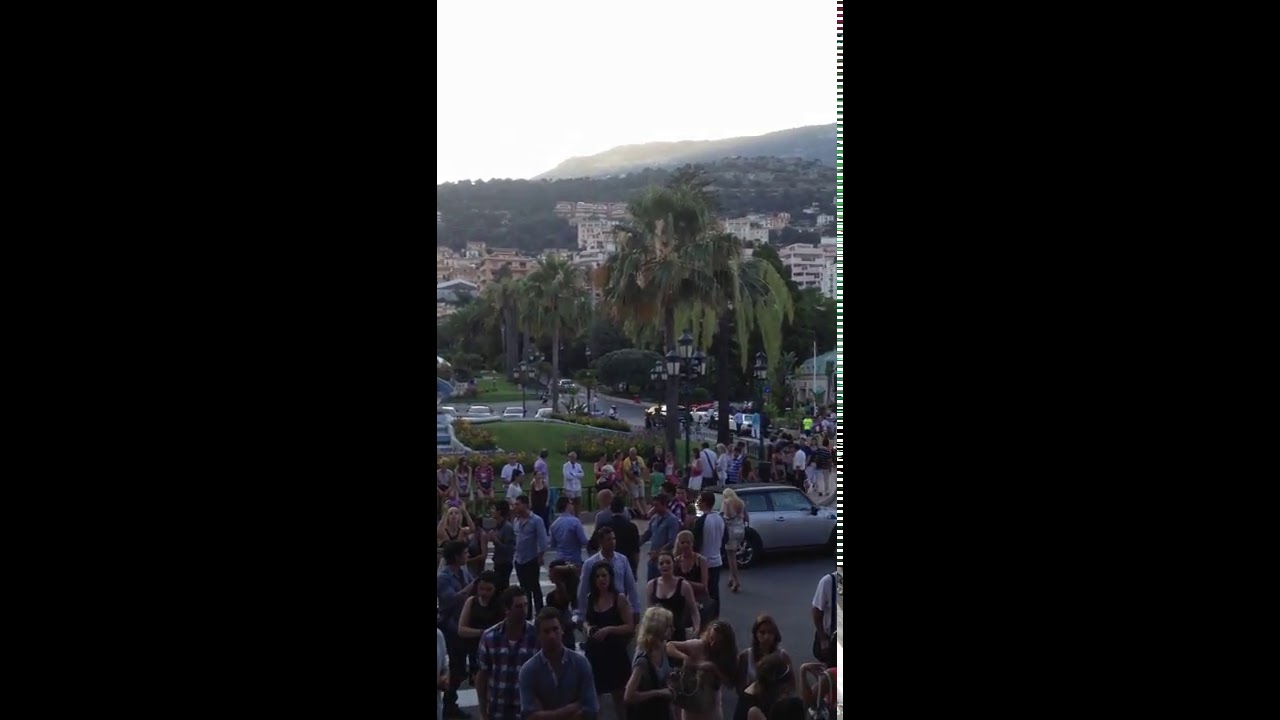In the foreground of this outdoor scene, a large and diverse crowd is gathered, composed of people in various colorful attire, including black, blue, white, checked, striped, and plain shirts. Amongst them, some women are seen in sleeveless dresses, and men predominantly in buttoned-up shirts. A small grayish car is also visible among the crowd. There is a dog interacting with its owner at the front of the image. 

The gathering appears to be taking place in a park, characterized by a lush green lawn surrounded by palm trees. Beyond the palm trees, there are white buildings and homes that ascend into hills in the distance. The sky behind the highest hill is pale and washed, indicating that the sun is setting. Additionally, a street lined with more cars and palm trees is notable in the background. The overall setting suggests a public event happening in the middle of the day, with a variety of colors—green, white, tan, purple, pink, yellow, and lime green—prominent across the scene. The photograph is framed by dark borders on the left and right sides.